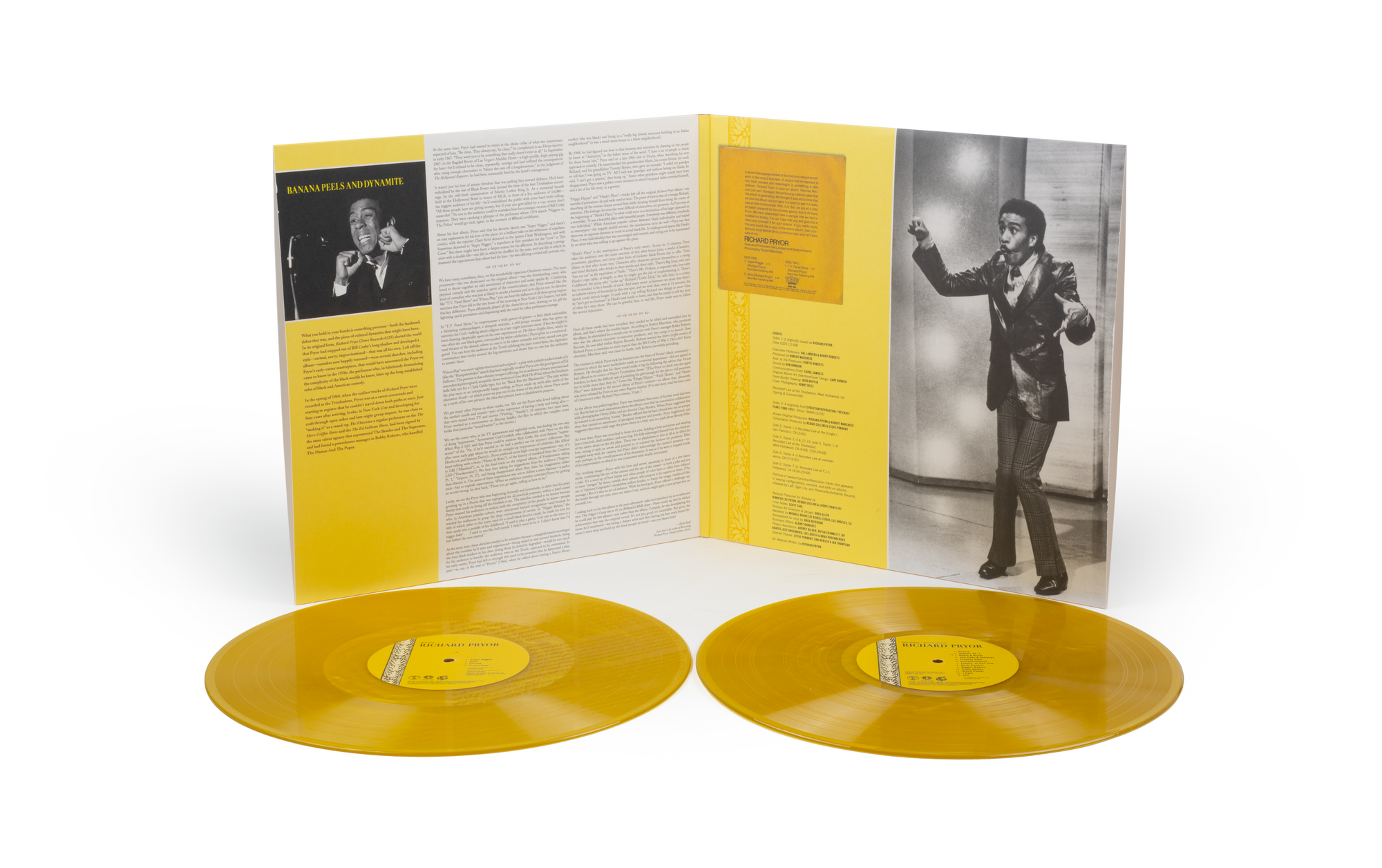The image depicts the inside of an open vinyl record album cover featuring comedian Richard Pryor. In the forefront, there are two vinyl records laid on a white surface, both colored in a mustard yellow with a matching yellow label at the center, marked by a gray strip. The label itself includes the name Richard Pryor and other details that are difficult to discern.

The album sleeve is opened like a book and prominently showcases two black-and-white photographs of Richard Pryor. On the right side of the sleeve, a full-length image captures Pryor in a dynamic stance with knees together, wearing a shiny jacket and plaid pants. His left hand is at his waist, while his right fist is clenched and raised in the air. His cheeks are sucked in, and his eyes are bulging wide, looking off to the left, reminiscent of a comedic pose.

On the left side of the sleeve, there is a square-cropped image of Pryor, along with extensive text that includes a section titled "banana peels and dynamite." The text, set on a yellow background, is largely unreadable in this particular view. Below this are additional paragraphs of text on a white background with black lettering. The entire inside cover is divided into sections with contrasting yellow and white fields filled with written content too small to read from the image.